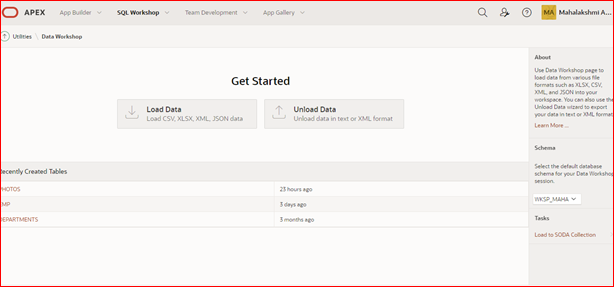The image displays a web interface related to Apex, as indicated by the label in the top-left corner. The main content area features a "Get Started" prompt with options to either load or unload data. On the right side of the screen, an 'About' section contains partially obscured text that includes "use data...page" alongside a visible red "Learn More" button and a word that appears to be "scheme."

A toolbar at the top of the page provides options for "App Builder," "SQL Workshop," "Team Development," and "App Gallery." Further to the right on the toolbar, there are icons for search, a user (person icon), a help section (question mark), and the initials "MA," which might refer to a user named "Mahakal Shawn A."

The main section of the screen displays a list titled "Recently Covered Tables," showing three entries with timestamps: one from 22 hours ago, another from one day ago, and the last from one month ago. Below these entries, a single task is listed as "Load to SC Collection."